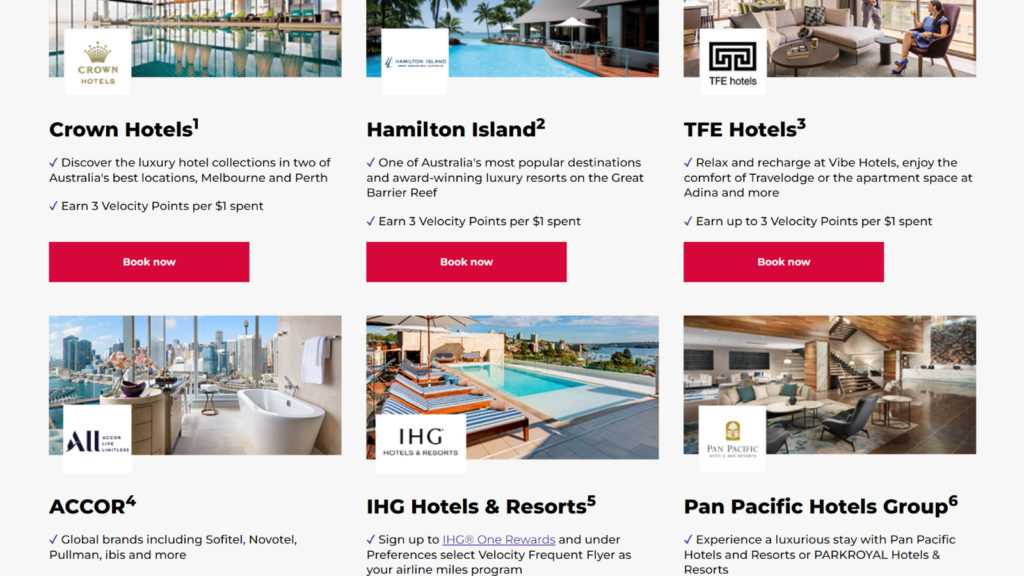The image showcases a travel website interface, possibly similar to platforms like Trivago, Expedia, or Hotels.com. The search results displayed on the screen feature six hotel listings. Each listing includes a hotel name and a "book now" button, although the bottom portion of the interface is cut off, obscuring the "book now" buttons for the latter three listings. The hotels listed are: Crown Hotels, Hamilton Island, TFE Hotels, Accor, IHG Hotels and Resorts, and Pan Pacific Hotels Group. Notably, the first two listings explicitly mention Australia, while the others do not specify a location. The search criteria appear to focus on luxury accommodations, as indicated by recurring mentions of luxury in the hotel descriptions.